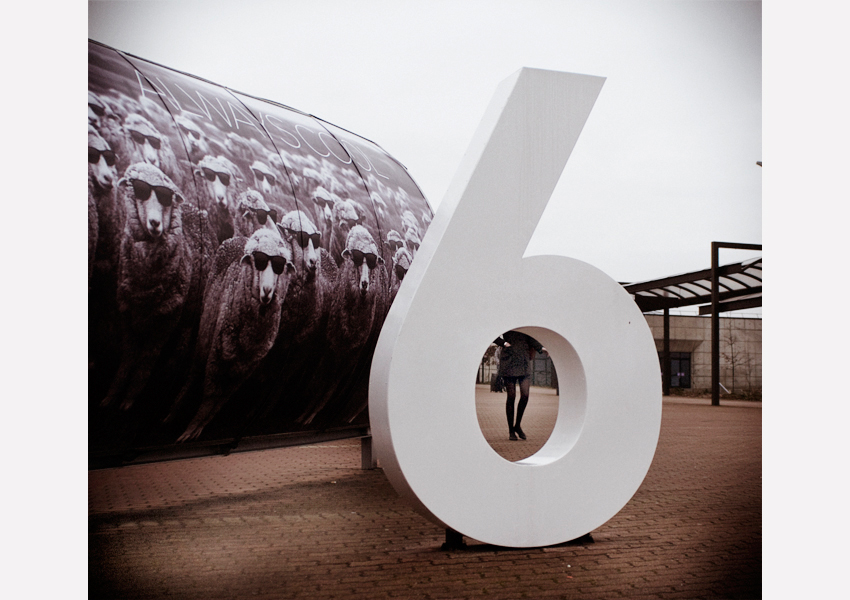This photograph captures an outdoor art installation set in a broad, bricked courtyard. The focal point of the image is a monumental white acrylic sculpture of the numeral six, standing upright and slightly tilted to the right. The hole in the center of the six frames the lower half of a woman walking towards the camera. She is dressed in black tights, black shoes, a black miniskirt, a gray jacket, and a black purse hanging at her hip. 

To the left of the six, a curved wall features the phrase "always cool" in white letters, under which a flock of sheep, all sporting sunglasses, are whimsically painted. The courtyard’s ground is paved with inserted bricks arranged in a zigzag pattern. In the background, a short, one-story building with a pavilion-like walkway extends outward, completing the scene under a white sky.